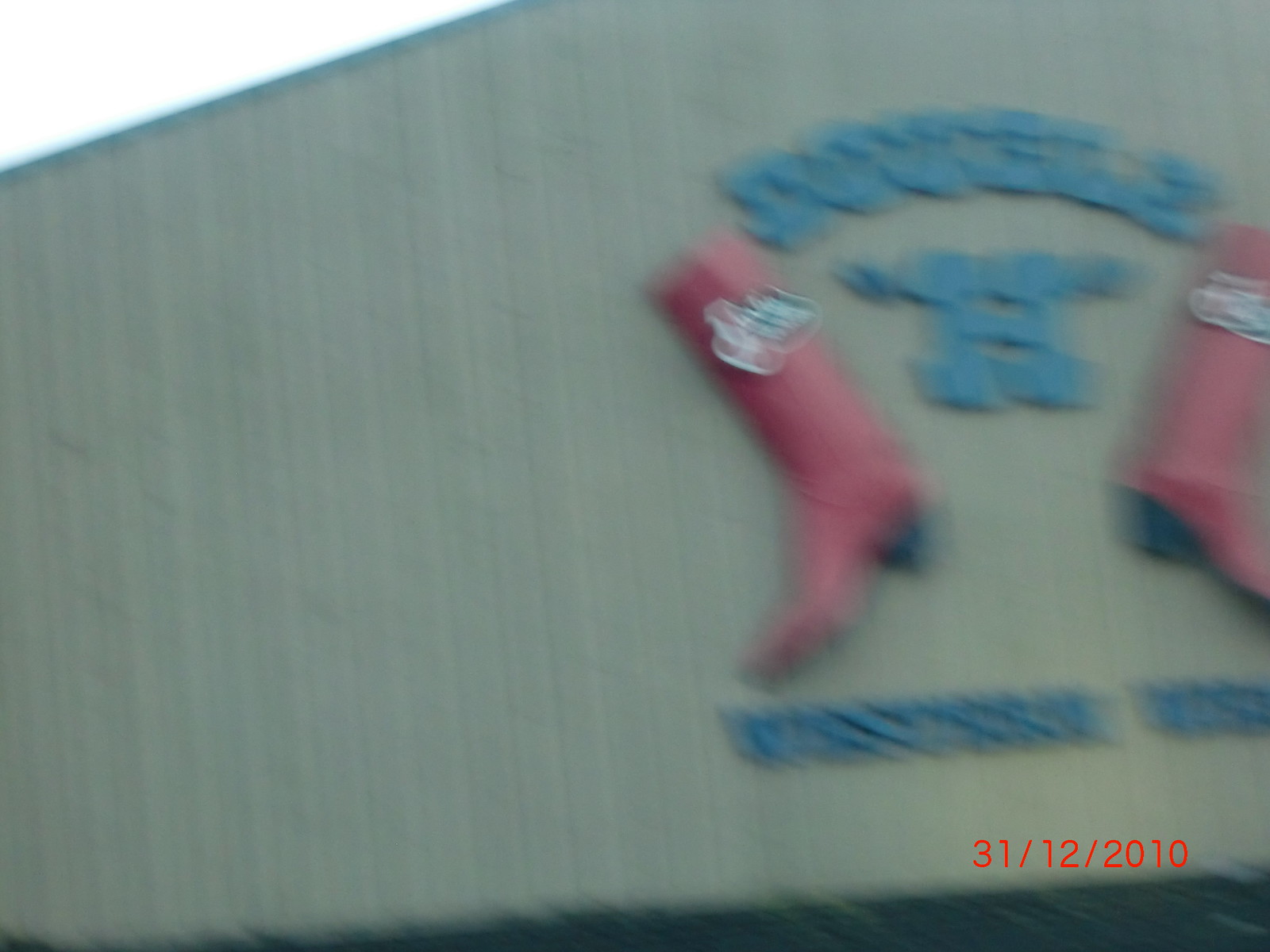This horizontal photograph, taken on December 31, 2010, captures an extremely blurred scene, making it challenging to identify details with precision. Dominating the upper right quadrant of the image is a pair of pink boots with black heels and soles, positioned diagonally from the center. The backdrop of the image features a light-colored surface, possibly a façade or wall, adorned with vertical lines or grooves that enhance its texture. Overlaid on this background, in indistinct blue lettering, is the name of a company, though the blurriness renders the text difficult to discern. The overall effect blends architectural elements with scattered footwear, creating an abstract visual narrative.